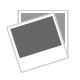The image showcases an abstract piece of modern art, primarily set against a predominantly white background that could be a canvas or possibly a white wall or curtain. Striking vertical dotted red lines cascade from the top to the bottom of the image, numbering around 20 or more, predominantly situated on the left side. The focal point features an intricate depiction that resembles a plant or flower with a dual-stemmed structure spreading diagonally from the bottom left to the top right. These stems, though not continuously connected, are rendered in black with various white lines and spots, giving them a wing-like appearance reminiscent of a dragonfly. The artwork is accentuated by a bright pink, oval-shaped splotch in the vicinity of what could be perceived as the flower’s petals, which seem to be closed and pine cone-like. Surrounding this pink area are numerous black and gray lines, adding depth and dimension. The entire piece is devoid of any text or signature, emphasizing its abstract and modernist nature.